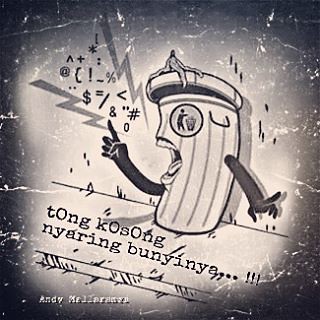This black-and-white hand drawing, likely intended as a public service poster or comic strip, features a central cartoon representation of a trash can with anthropomorphic qualities, positioned against a grayscale background that darkens towards the edges and lightens in the center. The trash can, depicted with arms and a large mouth full of teeth and lips, appears to be partially open, with a banana peel draped over its lid. The character is shown from a side profile, seemingly speaking in exaggerated frustration, indicated by a speech bubble filled with symbols and characters such as a dollar sign, slash, ampersand, at sign, and hashtag, commonly used to denote swearing or nonsensical speech. Surrounding the trash can are various foreign language texts, including illegible script above the can and additional writing on the sidewalk below it, contributing to the comic and somewhat chaotic atmosphere. This image possibly carries a humorous or educational intent, akin to a meme, highlighting the animated and expressive nature of the central trash can figure. Notably, the bottom left corner bears a signature reading "Andy" followed by an unclear surname.